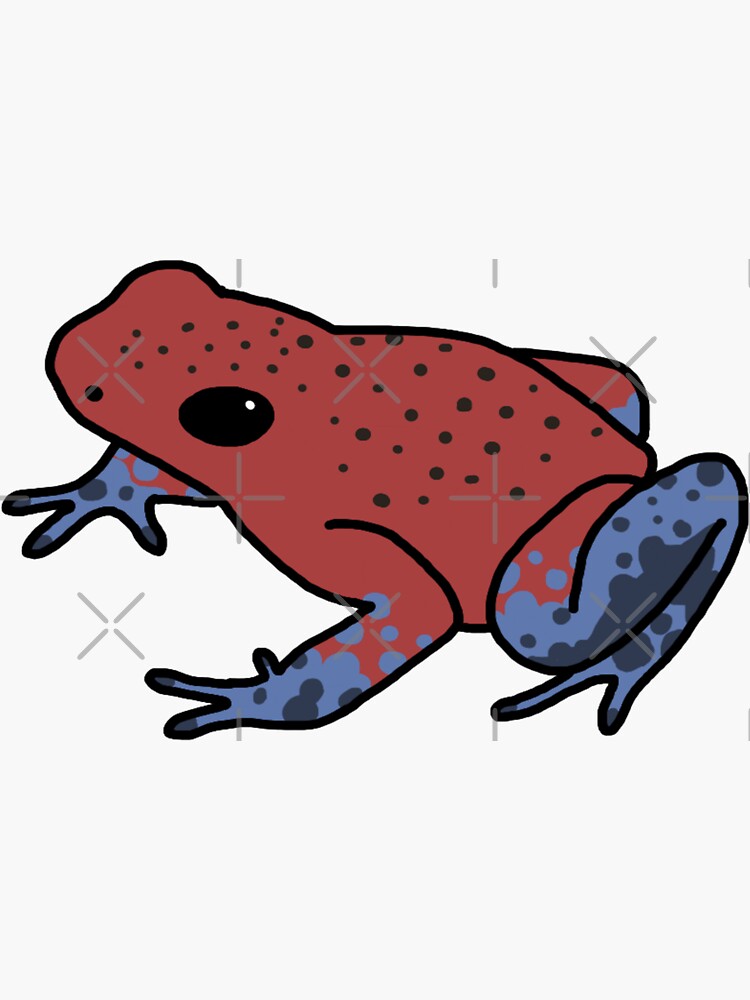This image is a detailed digital illustration of a whimsical tree frog set against a white background obscured by gray ink mark X's, suggesting an artistic or watermark purpose. The frog’s body is primarily a light reddish-brown with numerous black polka dots adorning its head and back. It possesses large, completely black beady eyes. The front and hind legs are mostly blue with tips in a darker shade, decorated with varying shades of blue and gray splatter effects and spots. The frog is positioned with its hind legs curled up and its front legs slightly spread out, showcasing webbed feet. The overall style of the image is cartoonish and resembles clipart, with distinct graphic elements highlighting the vivid colors and playful design of the tree frog.